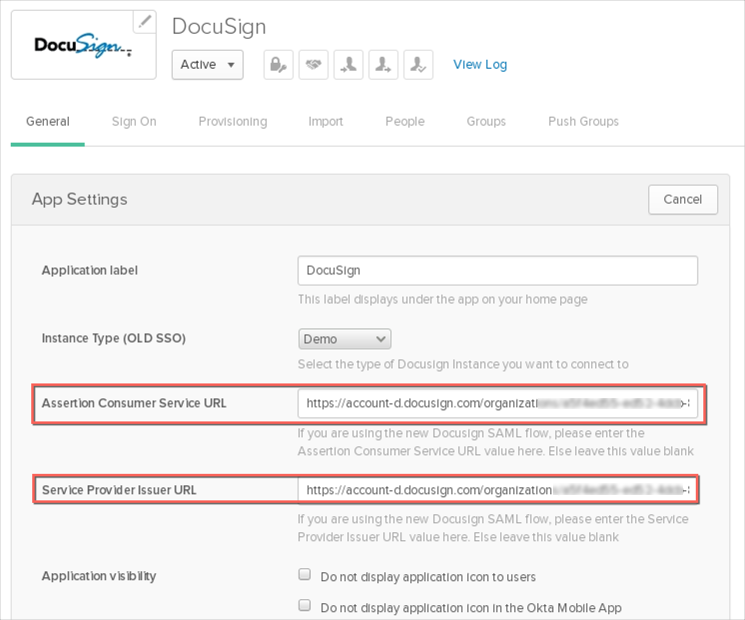The image depicts a DocuSign configuration page within an administrative interface. At the top, there is the iconic DocuSign text and logo alongside a drop-down button currently set to "Active." To the right of this are various other buttons, followed by a blue text link labeled "View Log."

Beneath this header, there are multiple tabs including: General, Sign-On, Provisioning, Import, People, Groups, and Push Groups. The "General" tab is currently selected.

Within the "General" tab, the page is divided into different sections. The first visible section is "App Settings," towards the right of which lies a "Cancel" button. Within "App Settings," the "Application label" has a text box populated with "DocuSign." Adjacent to this is a label, "Instant Type (Old SSO)," set to "Demo" via a drop-down menu.

Below this are two URLs entered by the user: "Assertion Consumer Service URL" and "Service Provider Issuer URL," both highlighted in red boxes, indicating they might need attention or validation.

At the bottom of the "General" tab's configuration section, under "Application Visibility," there are two checkboxes: "Do Not Display Application Icon to Users" and "Do Not Display Application Icon in the Okta mobile app," both of which are unchecked, suggesting the application's visibility settings are active by default.